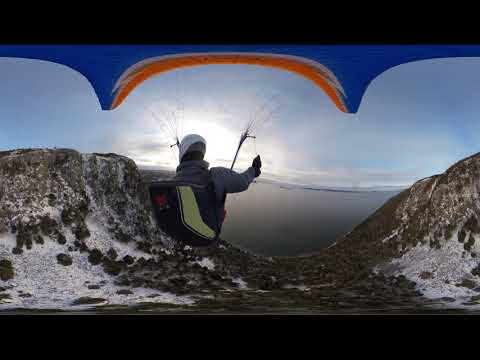A panoramic outdoor scene captures a person hang gliding, prominently situated slightly to the left of the center. The individual is securely seated in a black harness with yellow accents, sporting a gray jacket and a white and black helmet. Wires extend upwards, connecting them to a blue hang glider adorned with orange trimmings. The sky above is a vivid blue, scattered with a few clouds, and features a bright area near the person's head, hinting at the sun being obscured by some clouds. The hang glider soars over a picturesque landscape featuring tall, rocky hills with patches of snow and scrubby green vegetation. Below, the terrain varies from rocky outcrops to a gravelly valley, edged with patches of brown and gray detritus. In the distant middle of the image lies a large body of water, flanked by a distant shoreline under a cloudy, hazy horizon. Adding a dynamic frame to the scene, there are thick black borders at the top and bottom of the image.